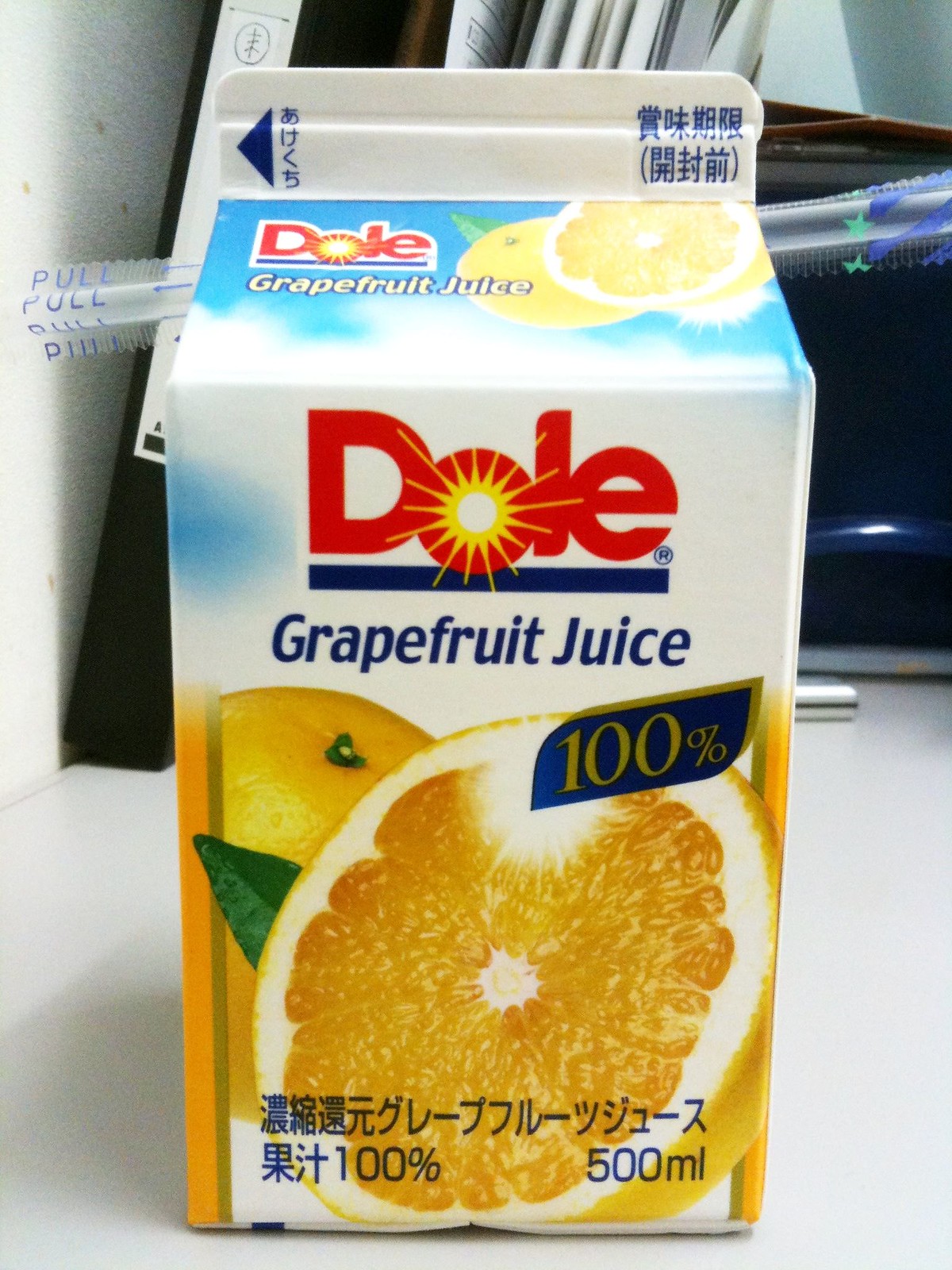This photograph captures a cardboard carton of grapefruit juice from the company Dole. Prominently featured on the carton is a 100% logo, signifying that the juice is made from 100% grapefruit. The majority of the text, including product details and nutritional information, is written in Mandarin characters, suggesting it is marketed towards an Asian audience. The carton is placed on a table, and a plastic straw is attached to its side for convenience. In the background, other objects are faintly visible, adding context to the scene. The bottom right of the carton displays "500ml", indicating the volume of the drink.